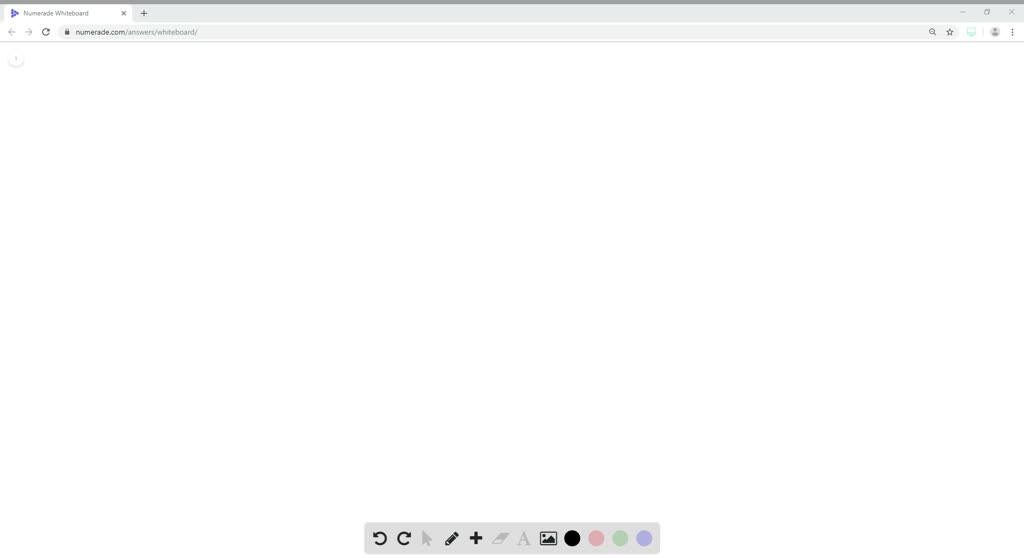Screenshot of a blank whiteboard webpage on Numerato, featuring a central white drawing area indicative of a typical online whiteboard used for collaborative purposes. At the top of the page, a search bar is visible. The bottom of the page showcases numerous control icons: a back arrow, a forward arrow, a pin tool, and a plus sign, among others that are indistinct. Additionally, there is an option to add photos, along with four color options for drawing or text (black, pink, green, and purple). This setup suggests tools designed for interactive group meetings and activities.